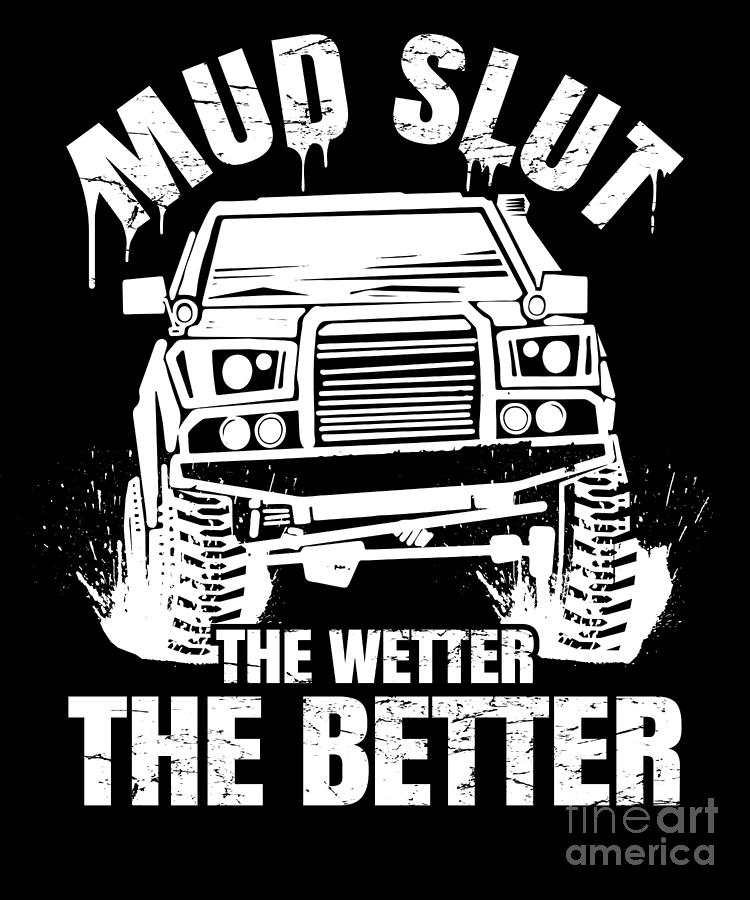The image appears to be a poster or flyer with a black background and features a striking graphic in white. Dominating the top of the image is the title "Mud Slut" in bold, white letters with a weathered, muddy appearance, accentuated by black splotches and dripping effects. Below the title, a large drawing of an off-roading vehicle with enormous wheels and prominent headlamps is depicted in white. The vehicle seems to be navigating through muddy terrain, with splashes of mud dynamically flying around it. The bottom of the image bears the phrase "The Wetter, The Better" in the same gritty, white text. In the bottom right corner, there is a semi-transparent gray watermark reading "Fine Art America," subtly overlaying the graphic's edge. The overall shape of the image is rectangular, with the length being twice the height.